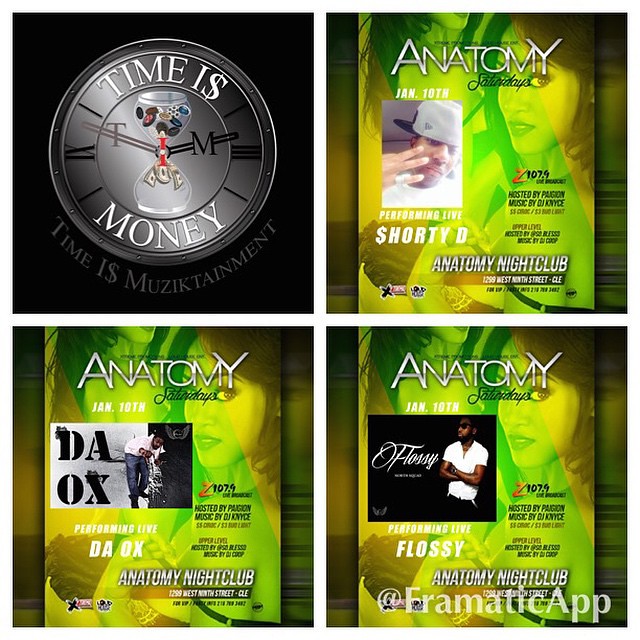The image is divided into four sections, laid out in a 2x2 grid. 

In the upper left section, there is a circular, black-and-gray illustration featuring an hourglass at its center. The hourglass has stacks of dollar bills at the bottom, and an indistinguishable object at the top. Encircling the hourglass are the words "Time is Money" in white text. 

The upper right section displays a green-tinted advertisement with a promotional poster for a nightclub named "Anatomy." The poster features the text "ANATOMY" in large silver letters and advertises a performance by "Shorty D," with the letter 'S' stylized as a dollar sign.

The bottom left section mirrors the promotional theme with another green-tinted poster from the same "Anatomy" nightclub. This poster announces a live performance by "The Ox."

The bottom right section also represents the "Anatomy" nightclub with a similar green palette, promoting a live performance by "Flossy." Each nightclub poster features promotional content relevant to distinct artists, along with dates in January for their performances.